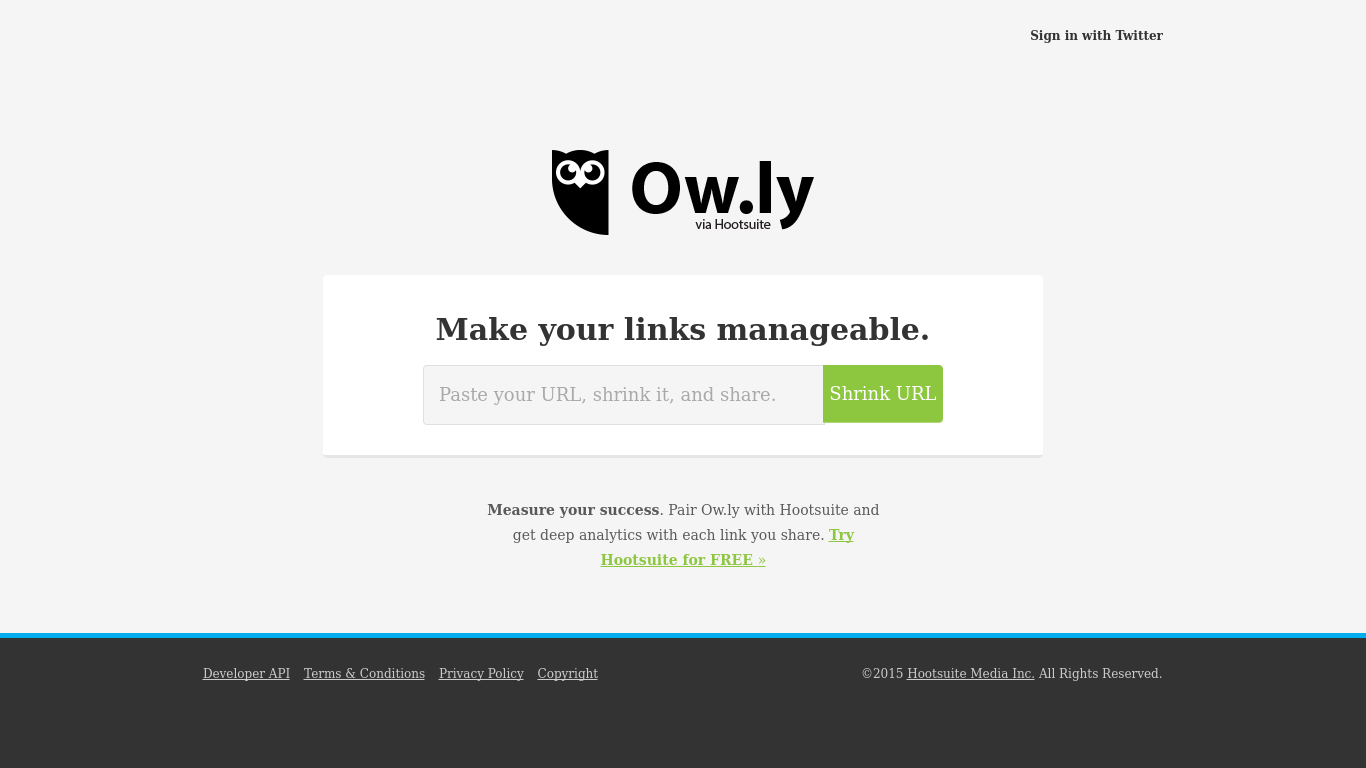Certainly! Here is a detailed and cleaned-up version of the caption for the image:

***

At first glance, the image appears to be a screenshot of a website designed for managing links. The background is predominantly white with black text. In the top-right corner, in very small lettering, there is an option to "Sign in with Twitter." 

The focal point of the image is an illustration of an owl, predominantly black with white outlines accentuating its eyes. This owl is named "Owly" (stylized as O-W-DOT-L-Y) as indicated by the small text beneath the image, which reads "via HootSuite."

Below the owl, there is a white box containing text that reads "Make your links manageable." Accompanying this is a text box inviting users to "Paste your URL, shrink it, and share," situated next to a prominent green button labeled "Shrink URL." 

Further down, the text "Measure your success" encourages users to pair Owly with HootSuite to obtain deep analytics for each shared link. This section concludes with the call to action, "Try HootSuite for free."

At the bottom of the image, there is a dark banner—possibly black or dark blue—containing several important links: "Developer API," "Terms and Conditions," "Privacy Policy," and "Copyright 2015 HootSuite Media Inc. All Rights Reserved."